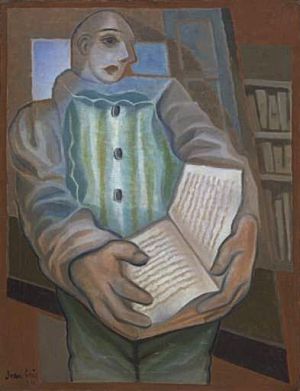This surrealist painting features a caricatured man with a disproportionately small, egg-shaped bald head and exaggeratedly large hands. He has pale skin and his face, reminiscent of a mime, has an unusual, distorted arrangement with a single right eye, directly below which is his mouth, flanked by an additional nose and a blank canvas on one side. The man is dressed in a striped teal suit with grayish sleeves and a button-down shirt adorned with dark buttons. He is holding an oversized book open, with pages featuring scraggly gray text. The background reveals a study or library setting, characterized by shelves filled with books, a counter, and an open window with blue shutters, set against a vibrant palette of red, white, blue, green, black, gray, peach, burnt orange, and tan. The painting is framed by a faint brown outline and is signed in the lower left corner, though the signature is hard to decipher.